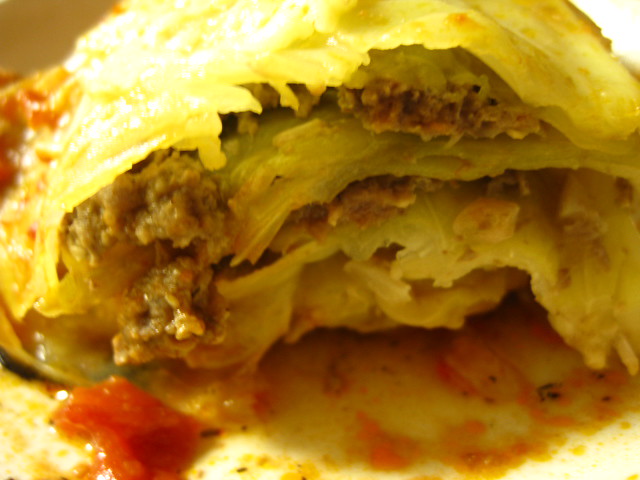This is a close-up, somewhat blurry and glare-affected photo of a food item that appears partially eaten, revealing its contents. The food in question could be a tortilla-based dish such as a burrito or taco, potentially even an egg roll due to its layered structure. Inside, there is a visible mixture of ingredients including ground beef or sausage, shredded or gooey cheese, lettuce, and pieces of tomato. The outer texture at the bottom closely resembles a tortilla, adding to the guess that it might be a form of Mexican cuisine. The gooey cheese runs along one side, enhancing the rich, layered composition of the dish.